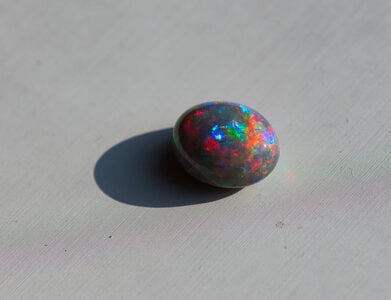This image captures a small, egg-shaped marble or gem, possibly an opal, with an electric, neon glow. The gem is decorated with an array of vibrant and brilliant colors—neon orange, green, blue, red, yellow, and pink—resembling a miniature galaxy. The surface of the gem displays both dazzlingly bright regions and patches of dark, muted tones where the light doesn't hit. A light source from the right side casts a distinctive dark shadow to the left on the plain, smooth, gray background. The overall simplicity of the composition emphasizes the extraordinary, colorful brilliance of the gem against its understated setting.